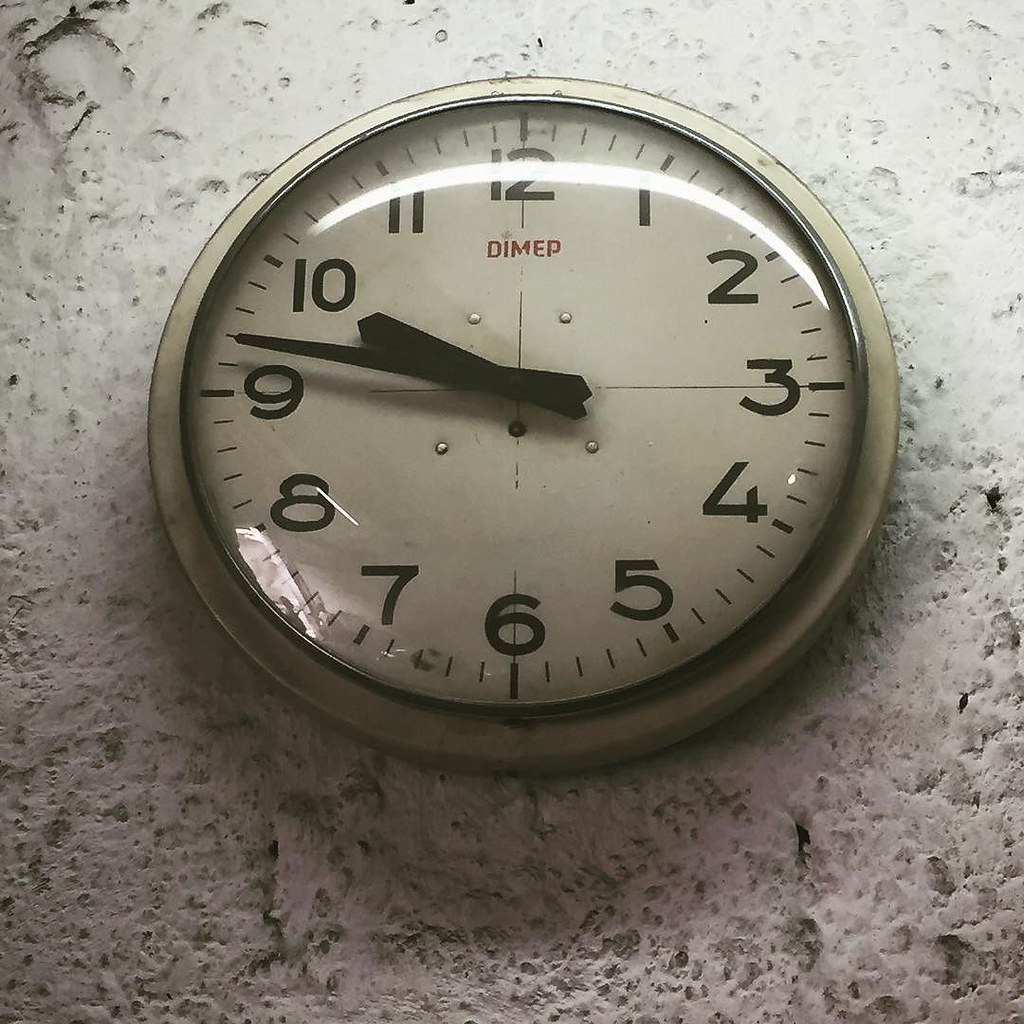This photo captures a vintage analog clock displaying the time 10:47. The clock, showing signs of age and wear, has a somewhat beat-up appearance. It features bold black numerals and black hour and minute hands, lacking a second hand. The clock face is encased in a silver bezel, providing a stark contrast against a rough concrete wall in the background. The once prominent brand name, "DIMEP," is faded and partially rubbed off in the center, hinting at its age. The overall style of the clock evokes a sense of nostalgia, reminiscent of the timepieces that adorned school walls in the 1980s.